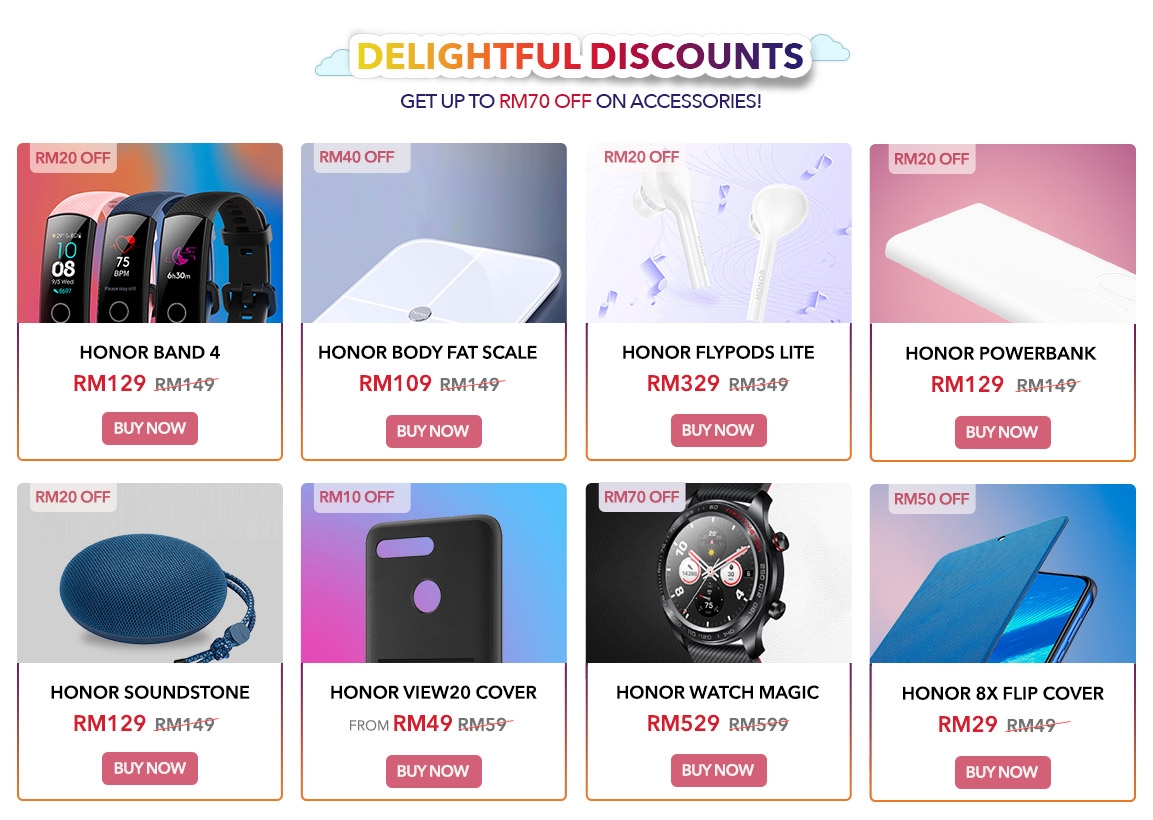This image depicts a vibrant online store or marketplace webpage. At the top of the image is a colorful title section adorned with clouds on both sides, drawing attention to the central text, "Delightful Discounts." This title is styled in a gradient color scheme that transitions smoothly from yellow to orange, pink, and purple, lending an eye-catching appeal. Beneath this, the text announces a promotional offer: "Get up to RM70 off on accessories."

Below the announcement, the page features two neatly organized rows, each containing four square tiles, showcasing various products. The first row displays the following items from left to right: an Honor Band 4, an Honor Body Fat Scale, Honor Fly Pods Light, and an Honor Power Bank. The second row presents an Honor Sound Stone, an Honor View 20 Cover, an Honor Watch Magic, and an Honor 8X Flip Cover. Each product tile includes a "Buy Now" button, indicating that the items are available for immediate purchase.